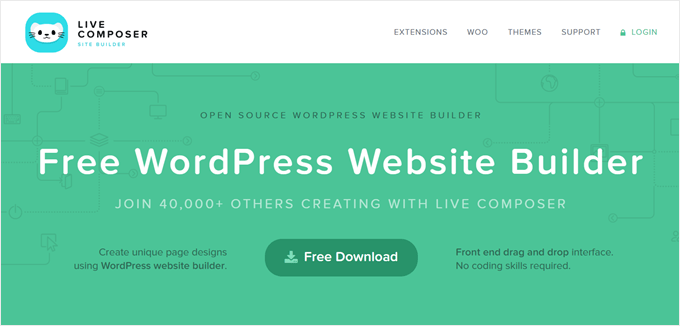A screenshot of a webpage predominantly features a cohesive and structured layout against a light green background with subtle, faded circuit board imagery. In the upper left corner, there is a blue box displaying a white mouse face with whiskers, ears, black eyes, a nose, and a mouth. To its right, the text "Live Composer" is prominently displayed, followed by several headers: "Extension," "Woo," "Theme," and "Support." In the upper right corner, there is a login option accompanied by a green lock icon, symbolizing security.

The main body of the webpage showcases a vibrant green section with contrasting black and white text. The heading "Open Source WordPress Website Builder" is written in black, followed by the large, bold white text "Free WordPress Website Builder." Beneath that, in smaller white text, it reads, "Join 40,000+ creating with Live Composer." Further down, the text, "Create unique webpage designs using WordPress and Mobile Builder," is displayed.

A prominent button labeled "Free Download," featuring a download icon to its left, invites users to take action. Below this button, another green box with white text states, "Front End Drag and Drop Interface, no coding skills required." The cohesiveness of the layout is enhanced by the elegant use of background imagery and clear, contrasting typography.